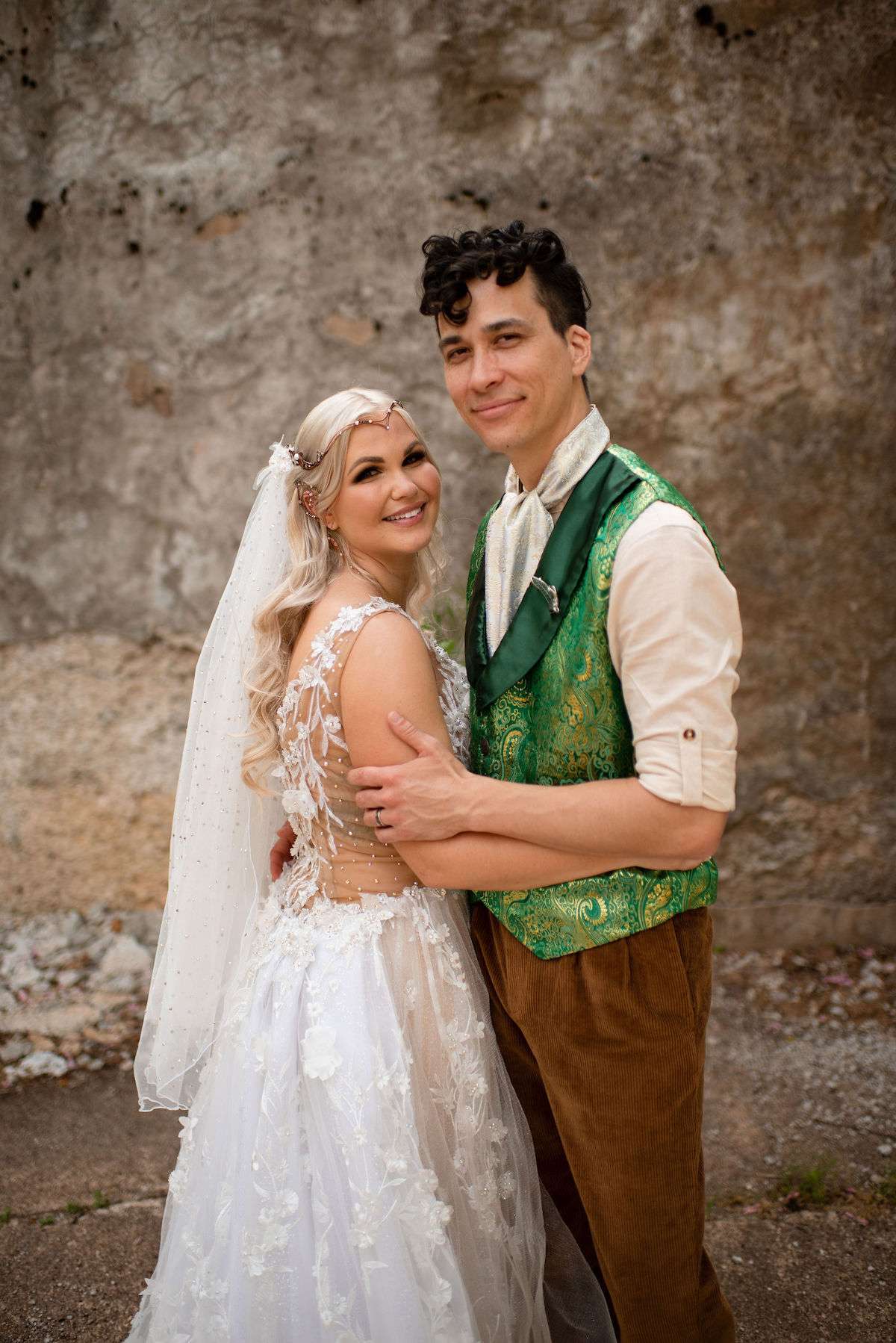This professional photograph captures an intimate moment between a newlywed couple. The man and woman are slightly embracing and smiling warmly at the camera. The bride, a smaller woman with blonde hair, is adorned in a white wedding dress featuring a delicate floral pattern at the bottom. A veil cascades from the back of her head, adding a touch of classic elegance. The groom, a man with curly dark hair, complements her attire with a white shirt rolled up to his elbows, a green patterned vest, and brown corduroy pants. He also sports a white ascot-like accessory. The couple stands in front of a gray and brown concrete or stone background, giving the image an industrial yet timeless feel. Their vintage attire evokes a sense of historical romance, reminiscent of the 1800s or 1700s. The overall composition highlights their joy and connection, making the photo a beautifully captured moment in time.